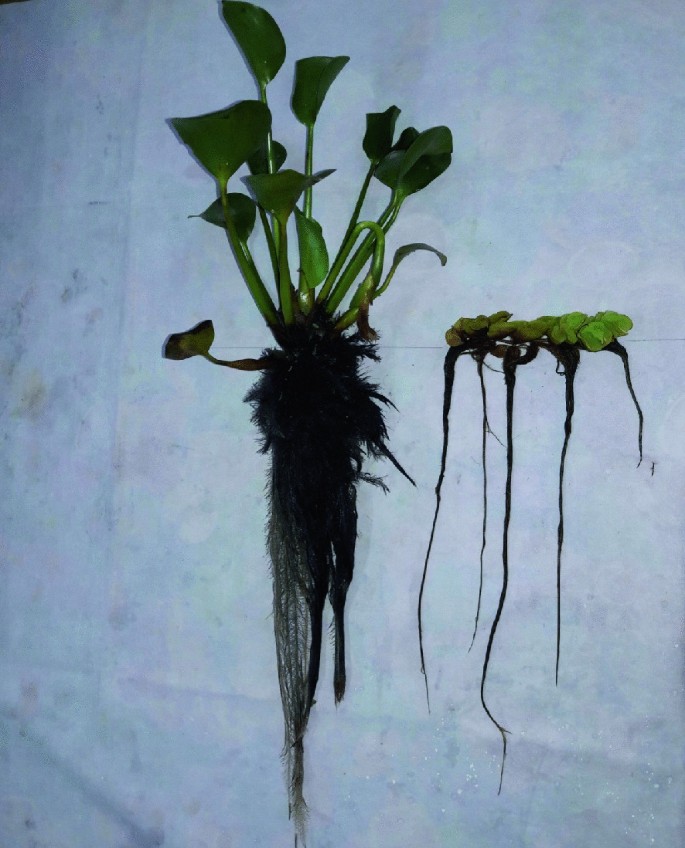The image depicts two uprooted plants laid on a crumpled white fabric, likely a cloth with visible creases. The white background serves as a contrasting backdrop. Both plants feature long, dirt-covered brown roots extending from their bases. The first plant is a cluster of cup-shaped, wrinkly petals or flat disks, resembling green aquatic plants with a mossy root structure, indicating they could be water plants. The second plant looks similar to a houseplant, potentially a pothos, with an impressive and extensive root system. The overall impression is that these plants were pulled out of a wet environment for closer inspection and photographic documentation. The photo itself appears aged and of low quality, adding a historical feel to the examination of these botanical specimens.